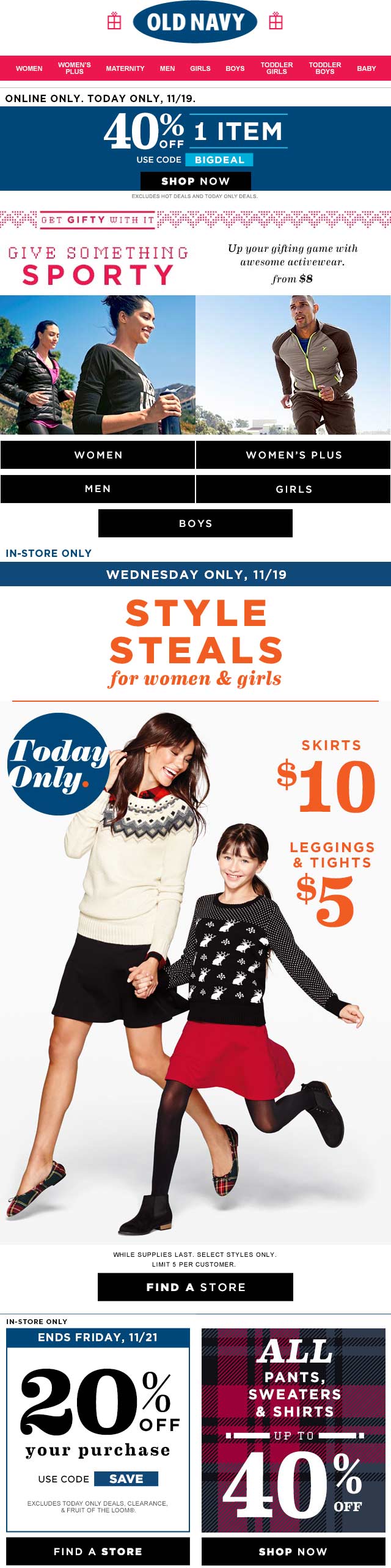This image is a screenshot from the Old Navy website, featuring a promotional banner. At the top, the iconic Old Navy logo is displayed in white text against a navy blue oval background. Below the logo, there are multiple navigation options for different clothing categories including Women, Men, Women's Plus, Girls, and Boys.

A prominent banner at the top announces a 40% off discount on one item, along with a promo code to use and a call to action to shop now. Further down, the headline "Wednesday Only, November 18th" catches the eye, accompanied by promotional details offering "Style Steals for Women and Girls."

The central image showcases an older woman and a young girl holding hands and running, embodying an active, joyous lifestyle. To the right of this image, more deals are advertised: skirts for $10 and leggings and tights for $5.

At the bottom of the snapshot, a button directs users to find a nearby store. Additionally, two discount coupons are displayed side by side: one offers 20% off your first purchase, expiring on Friday, November 21st, and the other offers up to 40% off on pants, sweaters, and shirts.